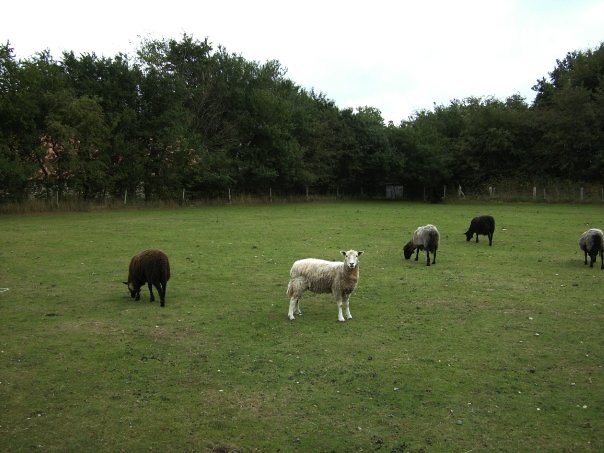This photograph captures a tranquil scene in a country setting during daylight. The expansive field, partly mowed down, is a mix of light green grass interspersed with brown patches and dotted with tiny white wildflowers. A hazy sky stretches above, predominantly gray with a sliver of blue visible in the upper right corner. Encircling the field is a dense line of tall, full trees that meet at a corner, with a faint, old wooden fence visible through the foliage.

In the field, five sheep of varying colors are present. At the center stands a white sheep, its gaze fixed directly at the camera, providing a focal point. To the left, a darker, possibly brown sheep grazes with its head down. On the right side, three more sheep—two grey and one black—are scattered, all with their heads to the ground, engrossed in grazing. The field exudes a peaceful, slightly gloomy ambiance, resembling a serene corner of a farm, perhaps reminiscent of a rural expanse in Ireland.